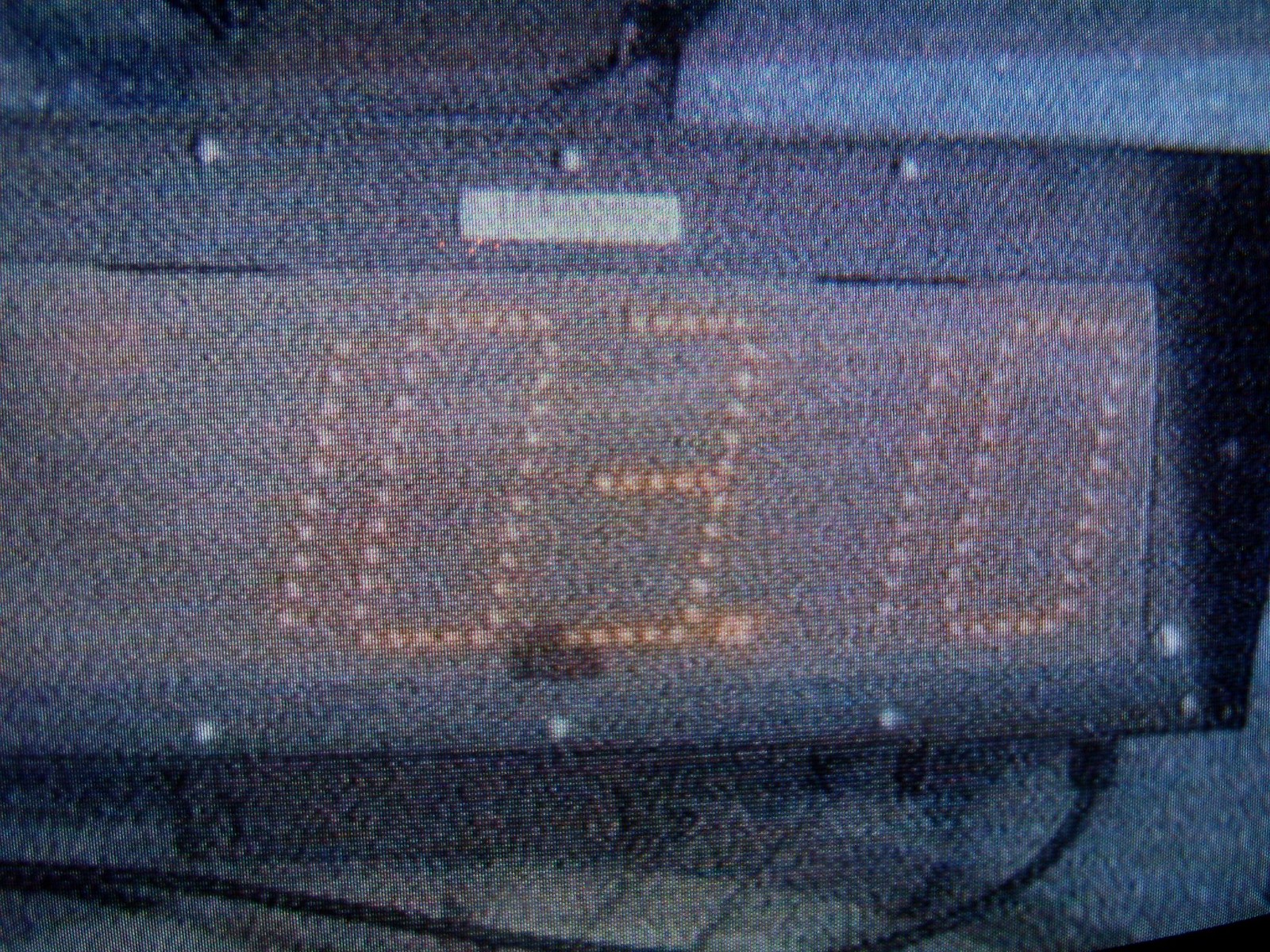The image showcases a close-up view of a clock radio encased in denim-like fabric. The background consists of the same denim material, creating a cohesive visual effect. The clock radio's surface is covered in this denim-textured fabric, although it's uncertain if it is authentic denim or a material designed to resemble it. The time display on the clock radio is illuminated in soft pink dots, clearly showing the numbers "103.10," indicating a radio station frequency. Surrounding the edge of the clock radio, there are small white dots, which appear to be securing the denim fabric to the device. Above the frequency display, there is a logo or symbol, but its details are indistinct and unreadable in the image.